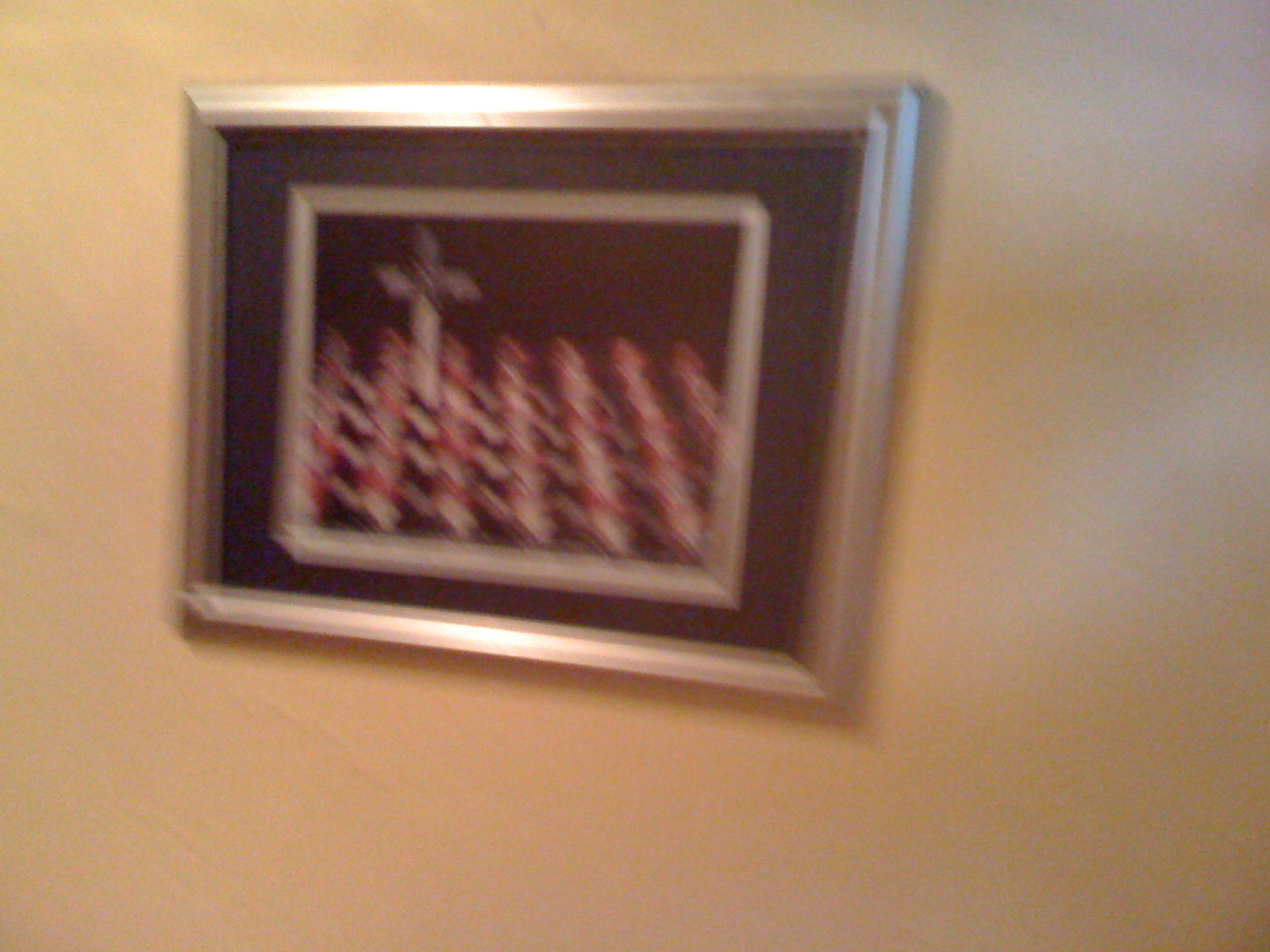In this image, we see a blurred photograph of a silver-framed picture on a beige or yellowish-white wall, which could be painted drywall or wallpapered. The frame itself has a black mat inside, which adds a stark contrast to the silver exterior. Within the frame, there's a photograph that primarily shows a silver crucifix located in the upper left-hand corner. Surrounding the crucifix, there is a grid-like pattern at the bottom, extending to the right. Additionally, there is an indistinguishable black item with a white top in the photograph, though its details remain unclear due to the motion blur. Light reflections are visible on the upper and bottom edges of the silver frame, and there is a noticeable drop shadow behind it. The background is nondescript, with no other items visible on the wall, and the photograph itself does not fill the entire frame, leaving portions of the black mat visible.